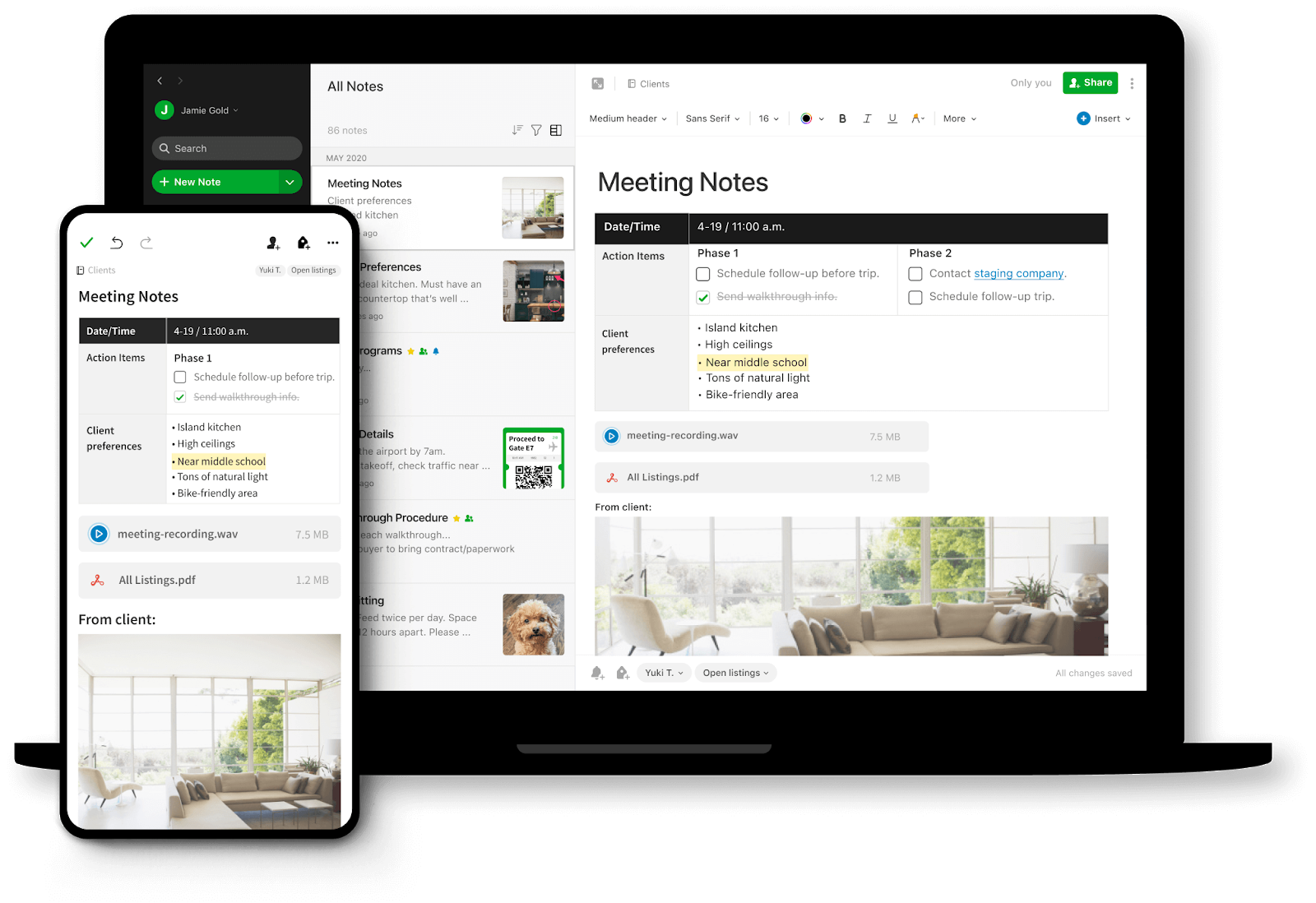A laptop and a smartphone are displayed side by side, both showing the same meeting notes. The laptop screen is centered with the smartphone on its left, each displaying a clear date and time for the meeting at the top. Below that, the notes specify action items divided into two columns labeled "Phase One" and "Phase Two," along with a section for "Client Preferences" featuring five bullet points. Both screens also indicate the meeting recording size as 7.5 megabytes and mention that a PDF of all listings is attached. At the bottom of both the laptop and smartphone displays, there is an image from the client depicting a living room or office area with a window, a chair, a sofa, and a couple of lamps. The caption concludes with a polite note thanking viewers for watching the webinar and inviting them to reach out with any questions for further assistance.